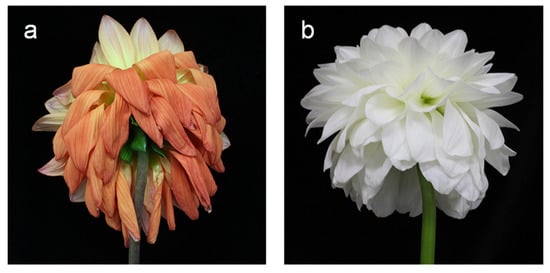The image consists of two square photographs of flowers set against a black background, positioned side-by-side. The photograph on the left, labeled with a small letter "A" in the upper left-hand corner, showcases a wilted flower with a combination of faded orange and white petals. The flower appears droopy, with a darker grey-green stem that adds to its withering appearance. Partially hidden white petals are also visible in the background. This flower might be a carnation but looks markedly different due to its wilted state.

In contrast, the photograph on the right, marked with a small letter "B" in the upper left-hand corner, features a vibrant white flower in full bloom with a flourishing, green stem. The white petals are delicate and abundant, giving an impression of health and vitality. Although it is not definitively clear if the flowers in both photographs are of the same species, their structural similarities suggest that they potentially are, showing two different states: one wilted and the other thriving.